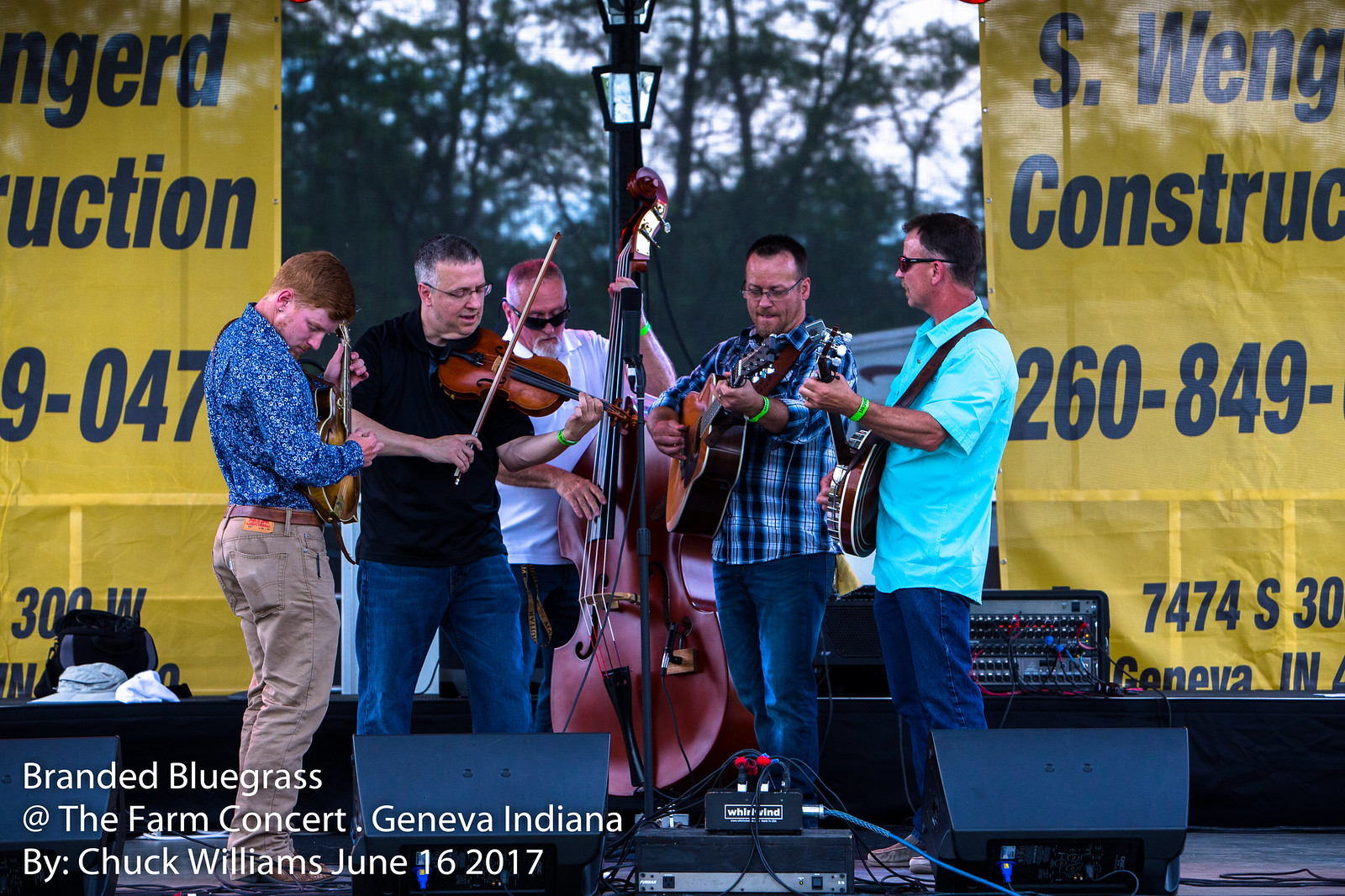The image portrays a lively group of five male musicians performing on an outdoor stage at the Branded Bluegrass at the Farm Concert in Geneva, Indiana, on June 16, 2017, captured by Chuck Williams. Each musician is engaged with his respective instrument: a large standup bass prominently in the middle, played by a man with glasses and a white shirt; to his left, a violinist in a black t-shirt and jeans; next to the violinist, a mandolin player in a flowery blue shirt and brown jeans with a leather belt; to the right of the bass player, a guitarist in a plaid shirt and jeans with an acoustic guitar; and at the far right, a banjo player. They stand behind banners, which are partially visible on the left and right, and an outdoor lamppost. The background reveals a serene setting with trees and daylight, enhancing the harmonious atmosphere of the concert. The stage is equipped with speakers and a web of cords, indicating a well-planned musical event.